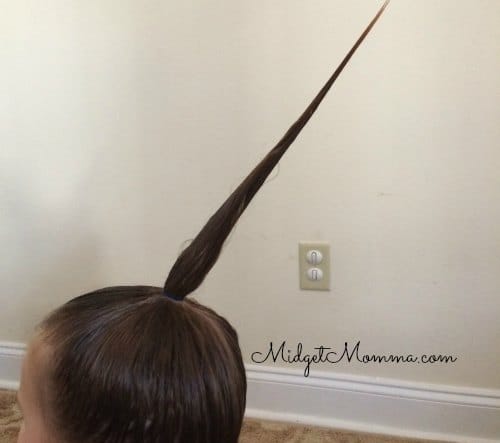In the image, a small girl, viewed mostly from the back and side, sits on a wooden floor next to a white wall with a beige outlet plate and white outlet covers. Her brown hair is styled into a pointed ponytail, held up by a small rubber band, which angles sharply upwards towards the right, almost reaching the top of the image. The wall forms the backdrop, while the outlet is centrally located towards the bottom of the image. The text "midgetmama.com" appears in cursive in the lower right corner. The setting appears to be a room within a house, possibly a living room, bathroom, or bedroom. The overall colors in the image are white, off-white, tan, and brown.